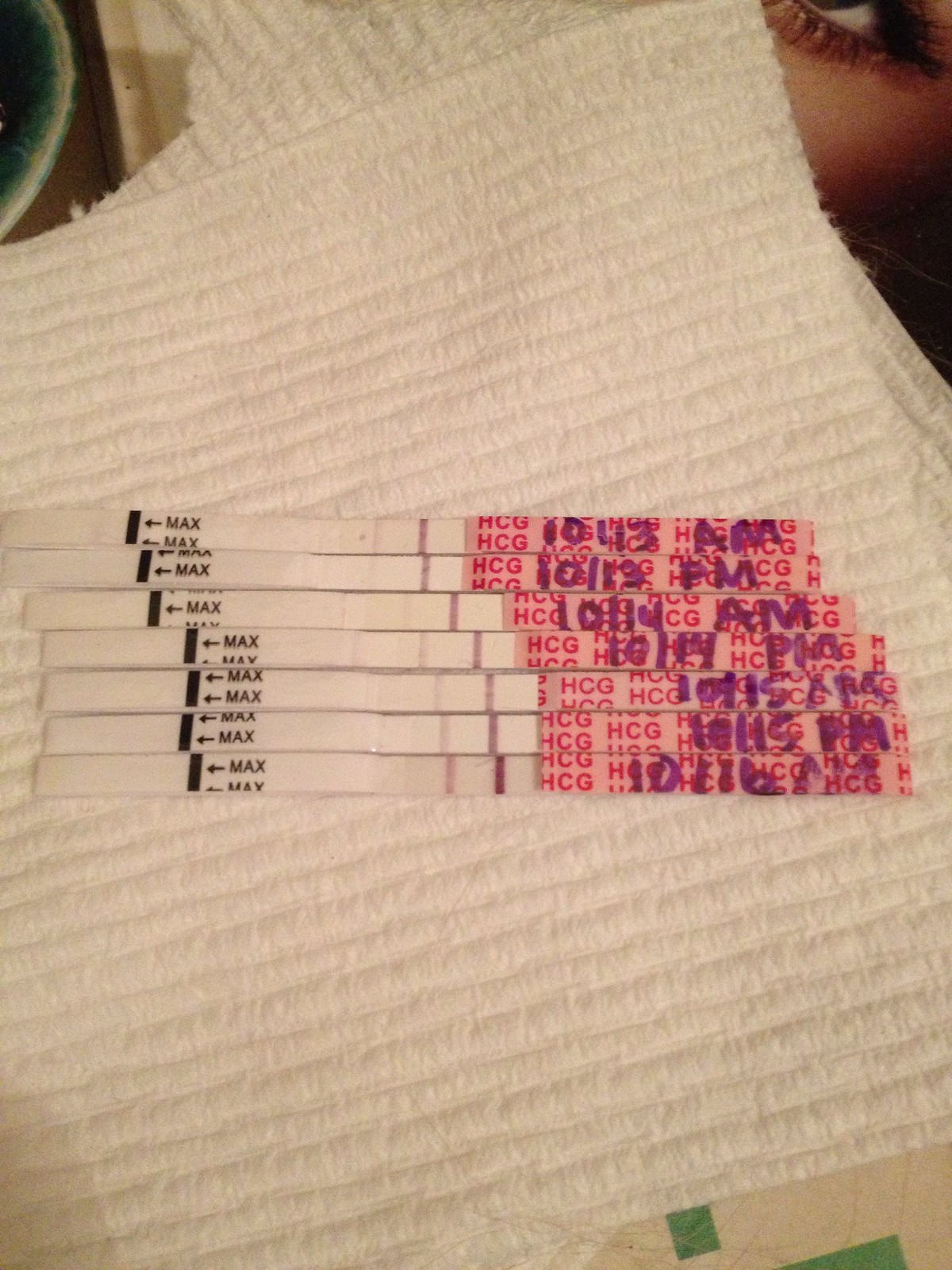In the photographic image, several pregnancy test strips are meticulously arranged on a white paper towel, which features a tear on one side but remains intact on the other. Adjacent to the paper towel, a green and white bowl—likely made of glass or ceramic—adds a pop of color to the otherwise neutral scene. A glossy magazine lies nearby, its cover showcasing a striking advertisement for mascara, featuring a close-up of a brightly made-up eye. Shadows cast along the edges of the photograph create depth and contrast. Scattered on the paper towel are a few strands of hair, subtly highlighting the daily life ambiance. The test strips, marked with HCG levels, display varying results; some indicate early testing dates with faint lines, while a dated strip from 10-11 prominently shows a much darker line, signifying a more advanced stage.